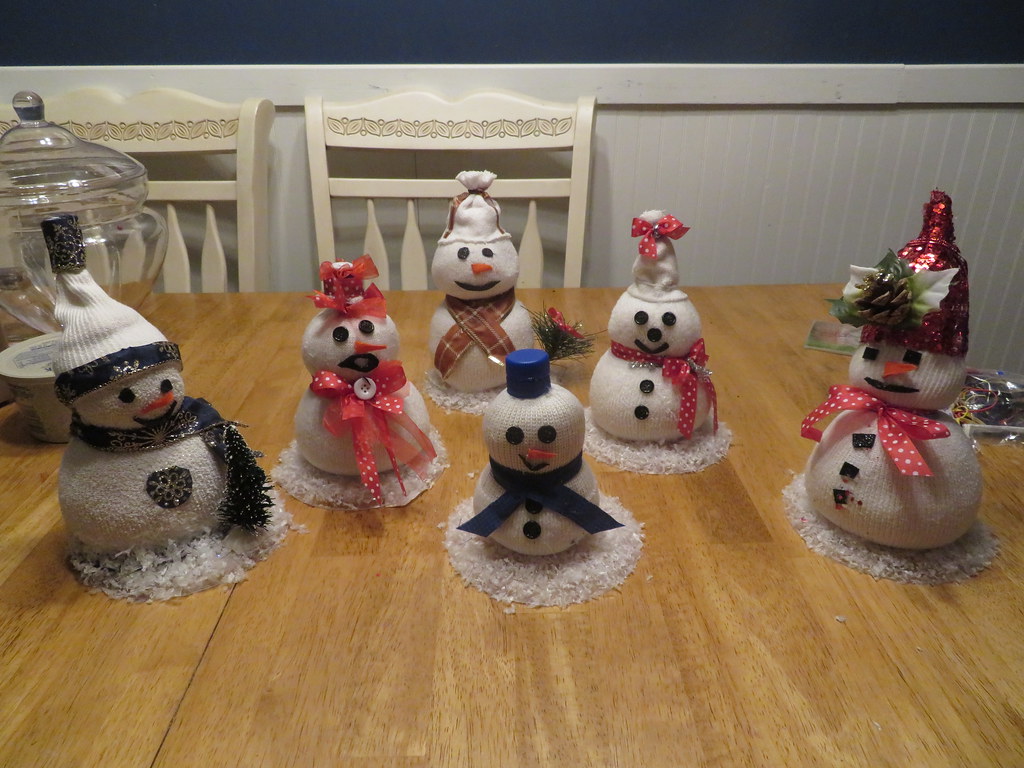A delightful Christmas-themed photograph showcases six handcrafted snowmen, carefully arranged on a light wooden dining room table. Each snowman, two balls high, appears to be made from various kinds of socks adorned with unique decorations, emphasizing their DIY charm. They are seated amidst a sprinkling of white confetti, creating the illusion of a snowy scene.

All six snowmen sport different hats and ribbons, adding to their individual personalities. The snowman on the far right is particularly eye-catching with its shiny red sequined hat, small pine cone with leaves, three irregular quadrilateral buttons, an orange pointy nose, a black mouth, and square black eyes. Next to it, a snowman features a red and silver accented bow around its neck, a white conical hat, and a small bow with a jingle bell at the top, notable for having a button nose instead of the more common carrot-like nose seen on the others.

In the center front, one snowman wears a cylindrical blue hat with a matching blue ribbon and two buttons on its chest. Behind it stands another with a white conical hat, adorned with a brown ribbon. To the left, a snowman boasts a small red conical hat with ribbons, an open black mouth, and a fanciful bow and white button on its chest. The far-left snowman completes the scene with a striking winter cap featuring blue and silver trim, a coordinating ribbon around its chest and a silver snowflake emblem on a blue circular background.

The table, likely in a kitchen, is flanked by two cream-colored chairs with white wooden slats on their backings and a light brown horizontal design at the top. The snowmen, each standing no more than six to eight inches tall, exude a heartwarming, festive charm that fills the room with holiday spirit.